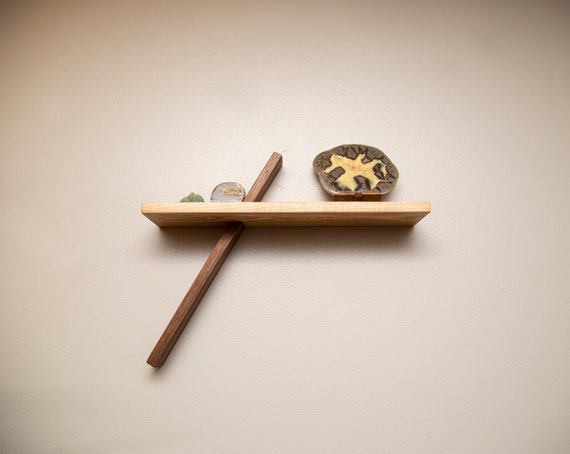The image features a small floating shelf made of light brown wood, attached to a cream-colored wall. This shelf is uniquely mounted by a diagonal, square-shaped wooden peg that goes through it from top to bottom on the left side, anchoring it securely to the wall. On the shelf, arranged left to right, are three distinct objects: a small green rock on the far left, a round glass object resembling a snow globe in the center, and a large, circular fossil-like rock on the right. The fossil is dark brown with a yellow figure in the middle. Notably, there's a prominent shadow on the top left corner of the image, with more subtle shadows in other corners, indicating some directional lighting. The entire setup has an earthy, natural aesthetic, highlighted by the textures and colors of the wooden shelf and the geological specimens it holds.